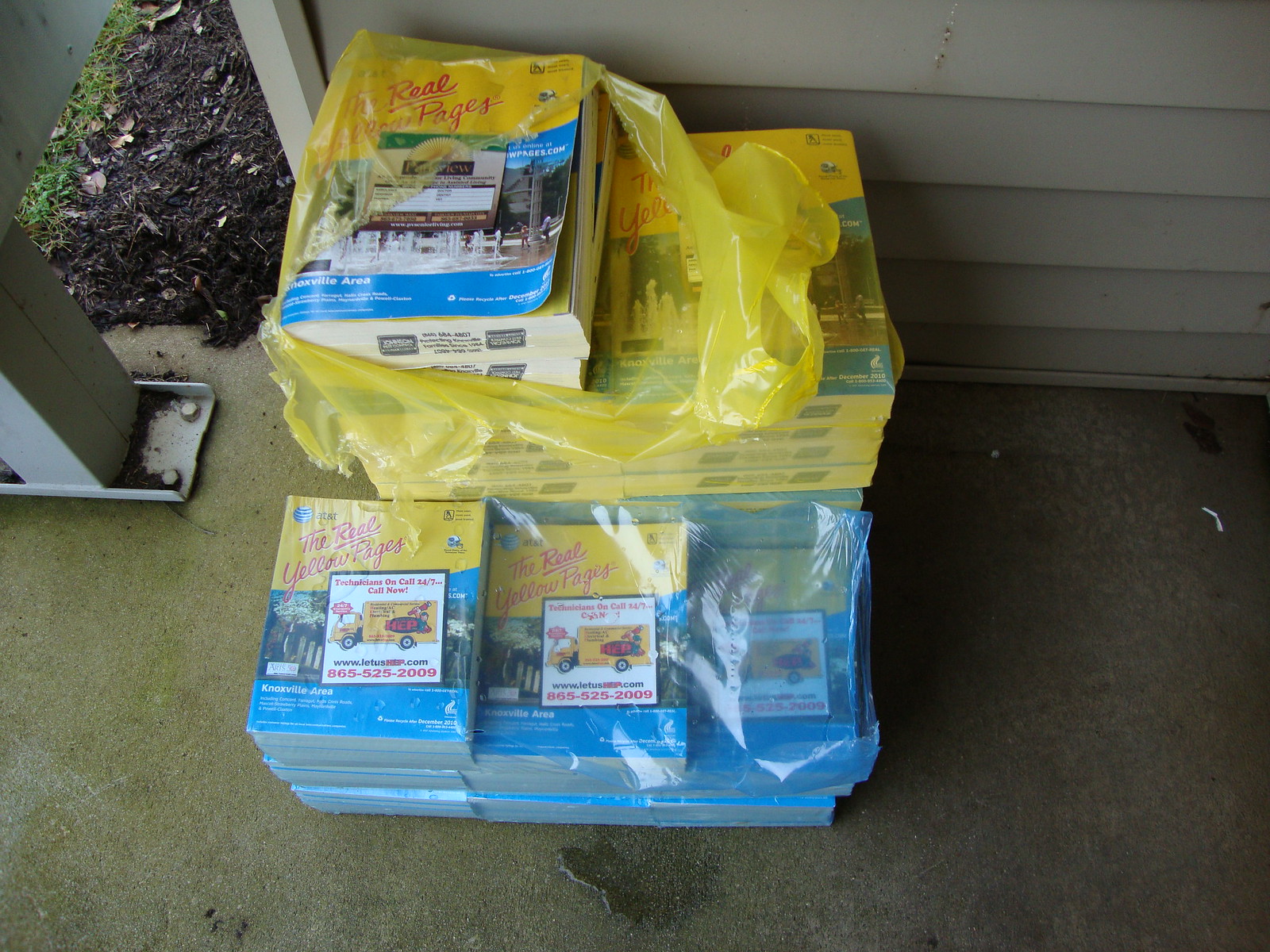The image depicts shrink-wrapped stacks of Yellow Pages telephone directories, sitting on a concrete porch with gray or beige aluminum siding in the background. The stacks are arranged with one shorter stack in front, wrapped in clear plastic, and a taller stack behind, wrapped in yellow plastic. The directories inside the yellow wrap have covers that are yellow at the top with the phrase "The Real Yellow Pages" (with "real" underlined), featuring various photographs which include images of buildings and a yellow bus. The bottom of the covers features a blue bar. 

To the left of the stacks, there is a support beam or pillar anchored to the concrete slab, with a small area of bark mulch and dirt visible, suggesting a garden space without plants but some soil and possibly grass. The porch area shows signs of wear, with some discoloration and black marks on the concrete, hinting at dirt. Overall, the setting appears to be the front stoop of a residential house, as indicated by the visible siding and support pillar.